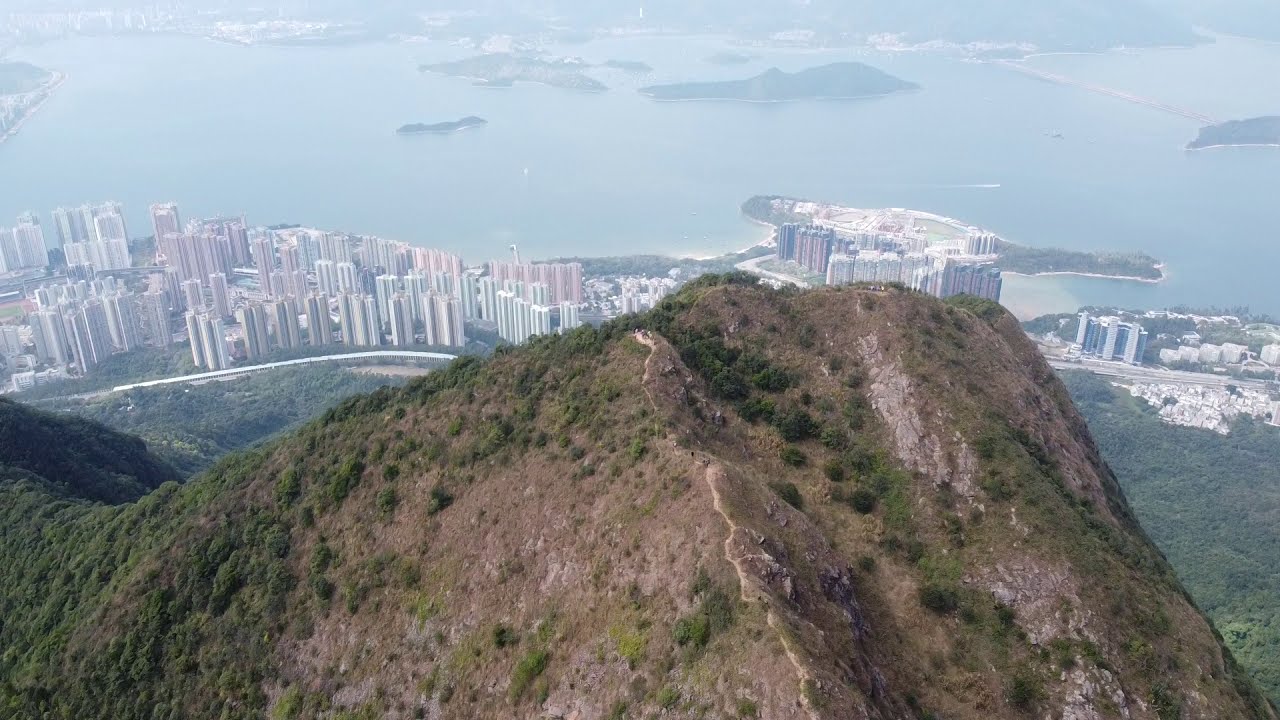This is an aerial view of a large mountain peak with rocky terrain, dotted with vegetation and dirt walking trails where a few people are visible at the very top. The mountain is significantly higher than the sprawling urban landscape below, which features a dense concentration of white and gray skyscrapers reminiscent of the New York City skyline. Beyond the tall buildings lies a vast bay with a noticeable collection of islands: three large ones and three smaller ones, creating a picturesque harbor. The water in the bay is a clear blue, contrasting the earth tones of the mountain and the greenish hues of the grass and trees scattered around. The city appears to be situated right on the water's edge and is bordered by more land and buildings in the hazy background. The diverse elements in this scene, from the towering mountain and winding paths to the bustling cityscape and serene bay, together create a captivating and detailed panorama.